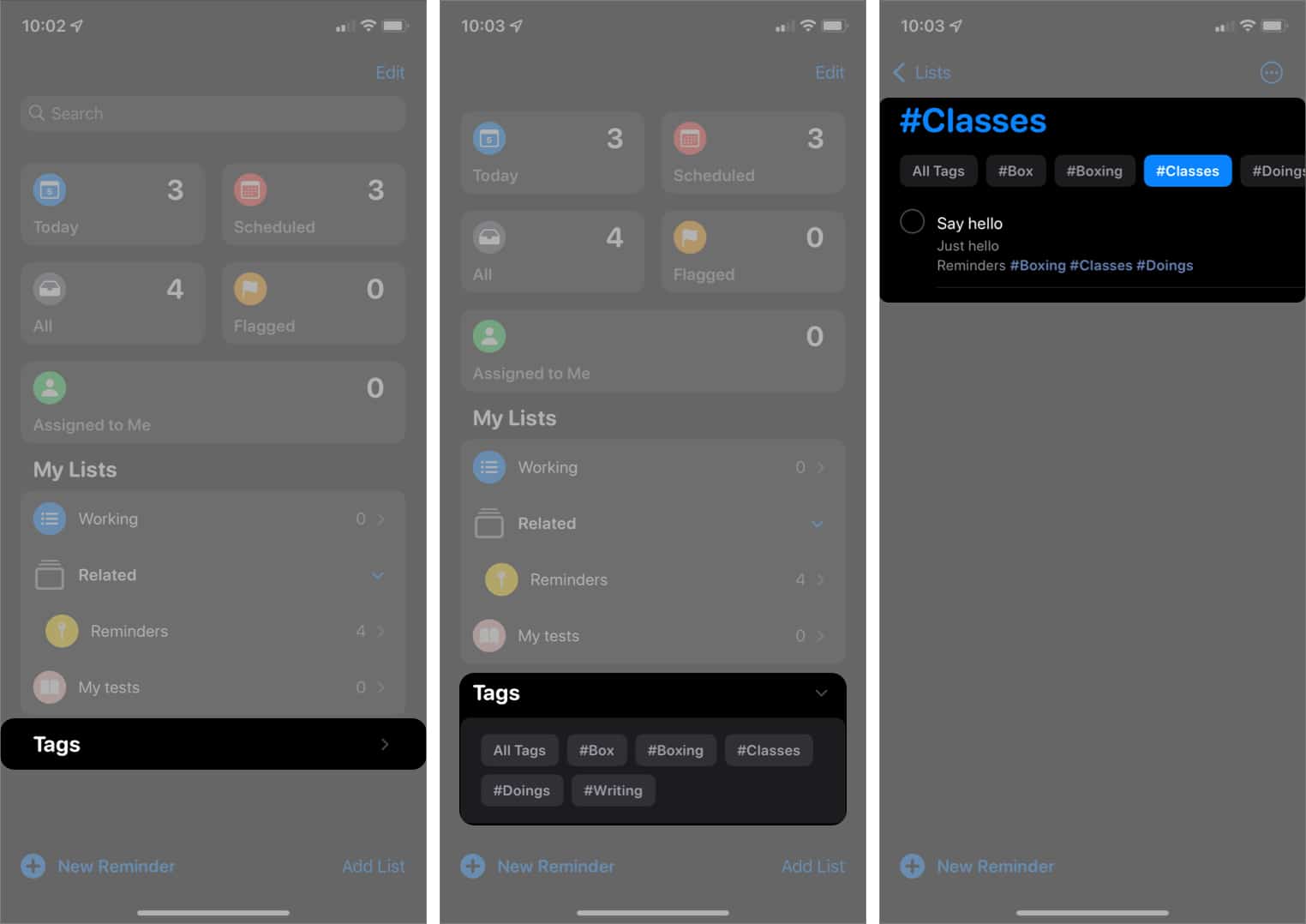Here is a detailed caption based on the voice description:

A series of three screenshots taken from a mobile device, each timestamped with different dates — "10-02", "10-03", and "10-03" from left to right. Each screenshot shows the device connected to Wi-Fi with two bars of signal strength and an almost fully charged battery. All screenshots have a uniform look, with a grayscale overlay indicating a highlighted portion of the interface. A blue circle with a plus sign labeled "New Reminder" is conspicuously located at the bottom left of every screenshot. 

At the bottom of the screen, a navigation bar is visible, featuring controls for going back and accessing the app drawer. The top right corner of the first two screenshots displays an "Edit" button, indicating an editable list or feature. 

The leftmost screenshot includes a search bar and a list of calendar-related boxes detailing "Today's Events," "Scheduled Events," "All Events," and "Flagged Events," each accompanied by a number indicating the count of events. Additionally, a section titled "Events Assigned to Me" features a blank profile picture icon in a green circle. Below this, the section "My Lists" with items labeled "Working Related Reminders" and "My Test" is displayed. A prominently black-highlighted portion with white text reads "Tags," followed by a forward arrow.

The middle screenshot mirrors the leftmost one in structure but extends the "Tags" section. It reveals that clicking "Tags" expands a dropdown menu with items such as "All Tags," "#box," "#boxing," "#classes," "#doings," and "#writing," each in a small grey box format.

The far-right screenshot focuses on the "#classes" tag, showing tags nested under it, including "All Tags," "box," "boxing," "classes," and "doings." Below these, in a smaller font, are items like "say hello," "just hello," "reminders," and hashtags including "#boxing," "#classes," and "#doings" grouped within the same box under the "#classes" tag.